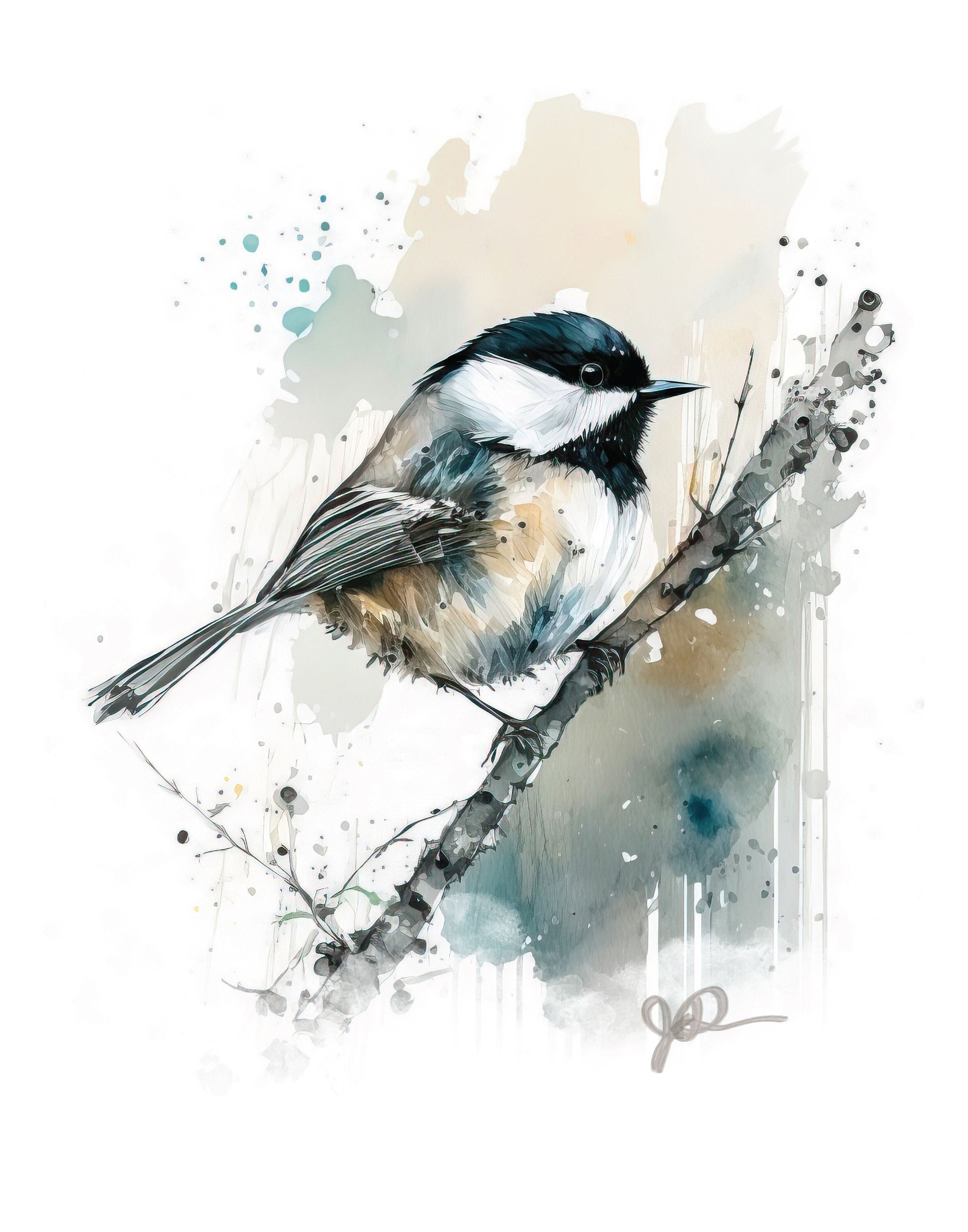This watercolor painting portrays a small bird perched on a twig, blending a harmonious palette of muted colors including shades of white, black, gray, beige, aqua, and blue. The bird, reminiscent of a chickadee, features a rounded head adorned with bluish-black feathers on top, a triangular patch of white feathers along the side of its face, and a pointed black beak. Its black eye is accented by a subtle white outline, adding a touch of delicacy to its gaze. The bird's body showcases a white chest and belly, with fine brown and beige shading near its bottom and sides, and distinctive black and white striped wings. 

The twig upon which the bird perches arcs diagonally from the bottom left to the upper right of the image, while the background evokes a serene, misty morning with blotches of gray, blue, green, and orange watercolor dots, enhancing the tranquil atmosphere of the scene. Amidst this dreamy backdrop, one can glimpse the artist's signature in gray at the very bottom of the painting, completing this beautifully detailed and soft portrayal of nature.